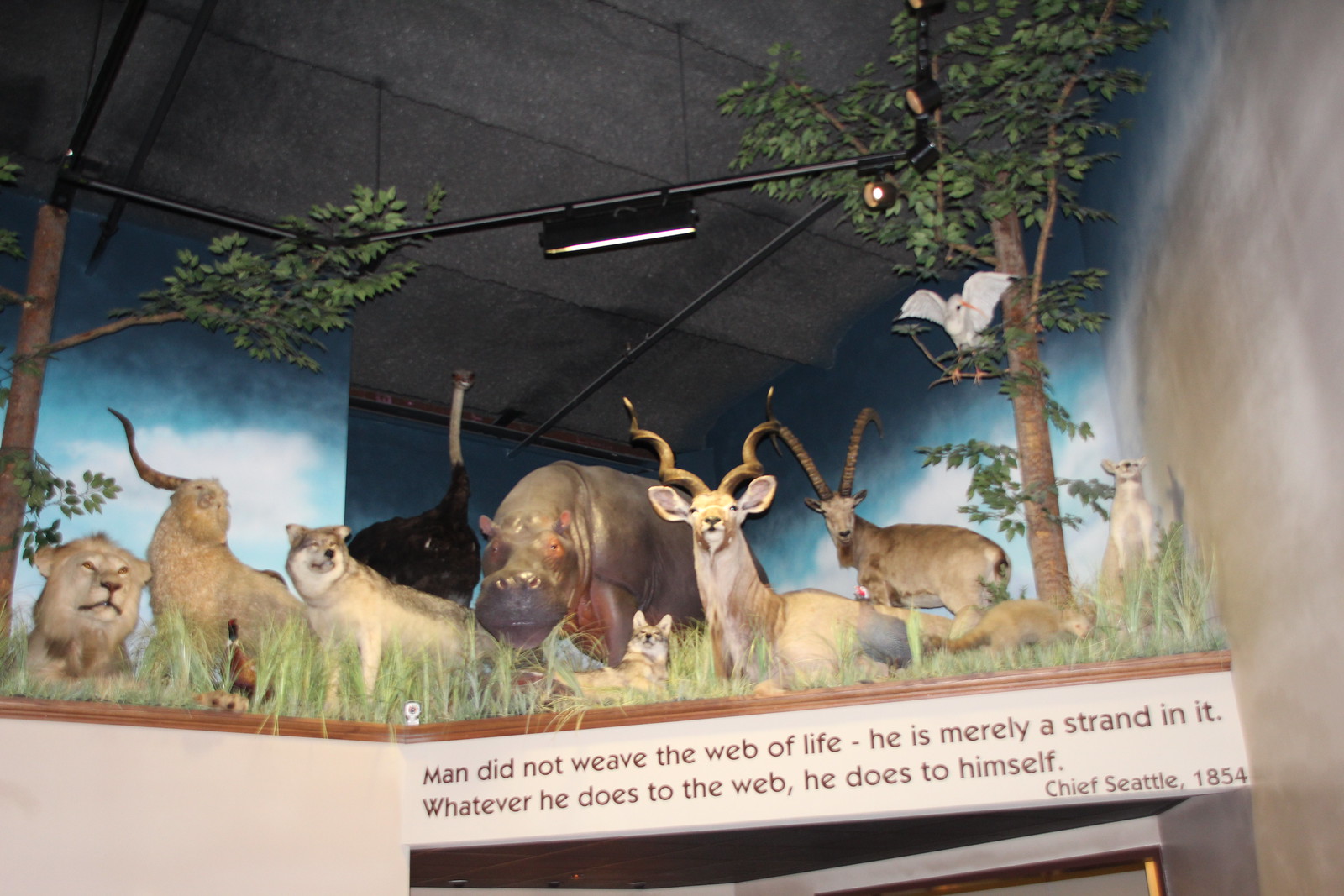The photograph, likely taken in a museum or an outdoor gear store, captures a dramatic display of taxidermied animals arranged above a blue, cloud-painted backdrop. Dominating the scene are a lion, a wolf, a hippopotamus, and an ostrich, accompanied by a gazelle or ibex, a deer, and a fox, among others. A white bird with a long beak nestles in a fake tree to the upper right, while another bird displays its outstretched wings in the foliage. Black metal track lighting is suspended from a grey ceiling, casting spotlights on the animals. Beneath the lifelike diorama, a quote reads, "Man did not weave the web of life, he is merely a strand in it. Whatever he does to the web, he does to himself. – Chief Seattle, 1854." A security camera discreetly watches over the scene, augmenting the museum-like atmosphere.